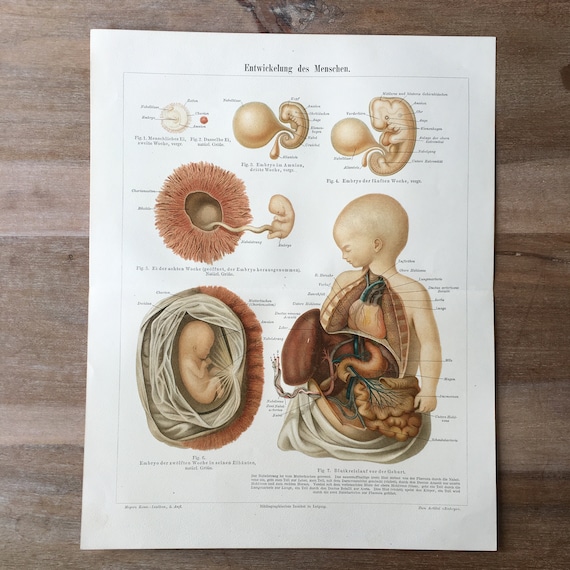This detailed caption describes an educational illustration of fetal development on a piece of white paper, likely sourced from a medical book or journal written in German. The illustration is divided into six distinct, colorized stages of development, from fertilization to a near-term fetus, all labeled in black ink. Starting from the top, the first image shows the fertilized egg, progressing through early stages where the zygote begins to form. Midway down, it illustrates the growing placenta and the enlargement of the fetus. On the lower left, there is a detailed depiction of the fetus within the womb, umbilical cord visible, surrounded by red shadings representing the uterine environment. The final, largest image on the lower right provides a cross-sectional view of the fully formed fetus, highlighting internal organs such as the lungs and stomach. This educational piece, laid on a wooden table for the photo, serves as a clear, labeled depiction of prenatal development stages from a single cell to a fully developed baby.